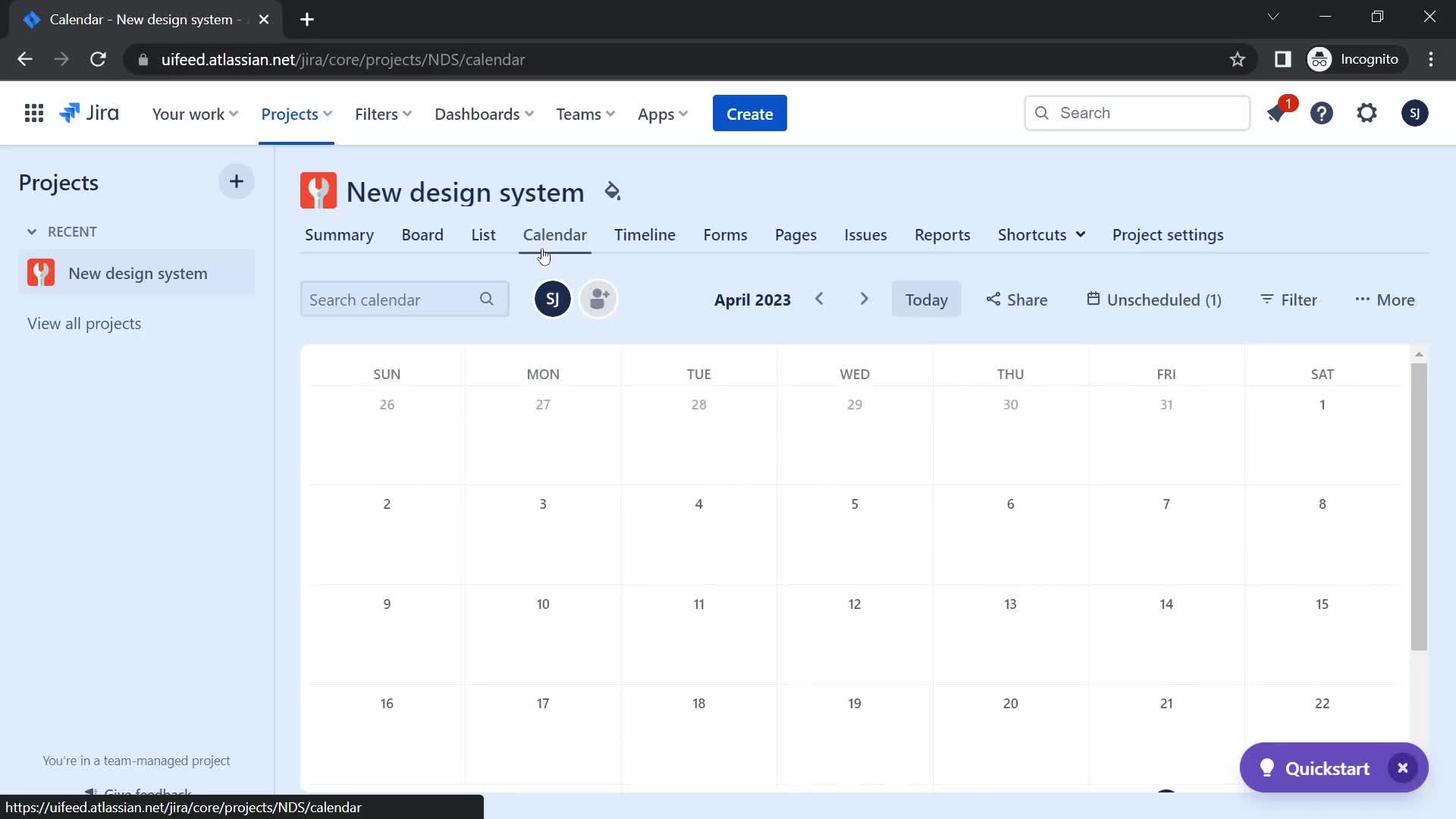This is a computer screenshot captured in April 2023, displaying a partial view of a digital calendar from a platform hosted on "jfeed.atlassian.net." The visible section of the calendar covers dates from the 1st to the 22nd, with a scroll bar indicating additional dates below. The interface showcases several navigation tabs, including "Your Work," "Projects," "Filters," "Dashboards," "Teams," and "Apps." A prominent blue "Create" button stands out, alongside a search box.

In the upper right corner of the screen, various icons are visible: an incognito mode indicator, a star, a notification bell with a red circle showing '1,' a question mark, a flower-shaped icon, and an "SJ" avatar probably representing the user's initials. There's also a wrench icon positioned at the top near the heading "New Design System." Finally, a vibrant purple "Quick Start" button is located in the bottom right corner, suggesting an option for rapid navigation or initialization of a task.